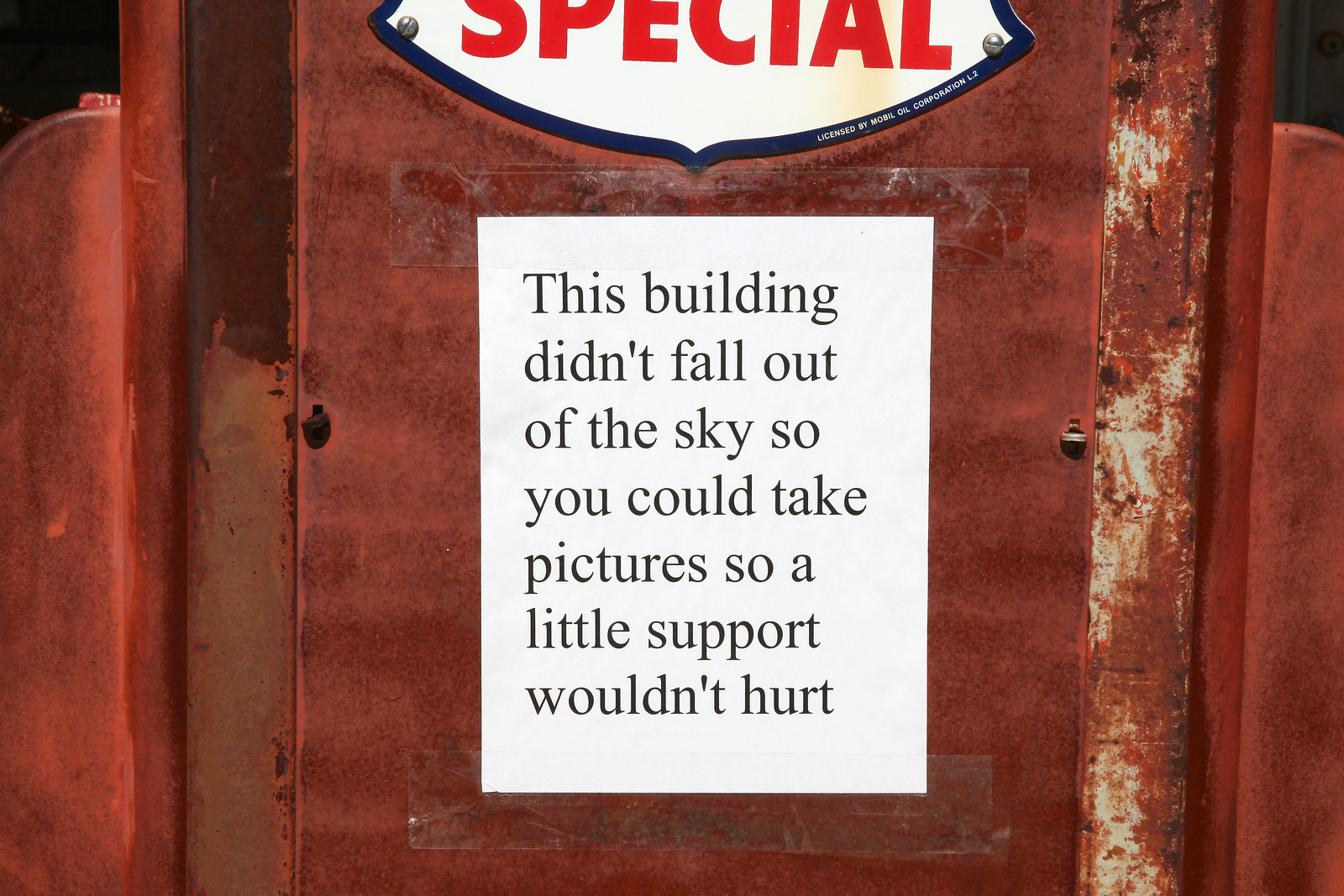The image depicts a close-up, high-quality photograph of a rusted, red metal surface, possibly part of an old gas pump or a dilapidated metal building. The metal surface is heavily rusted, with areas where the red paint has almost completely corroded through. Affixed to this weathered backdrop is a white piece of printer paper taped to the surface, featuring a bold, black printed message that reads, "This building didn’t fall out of the sky so you could take pictures so a little support wouldn’t hurt." Above this makeshift sign, there is a riveted, possibly bell- or lemon-shaped metal plate, labeled "Special" in red lettering. This plate also features a fine print along a blue edge indicating "licensed by Mobile Oil Corporation L2." The corners of the image sink into darker areas, suggesting the object extends into shadow or an incomplete frame. The overall appearance of the scene conveys a sense of abandonment and decay, with a somewhat paradoxical plea for respect and preservation.